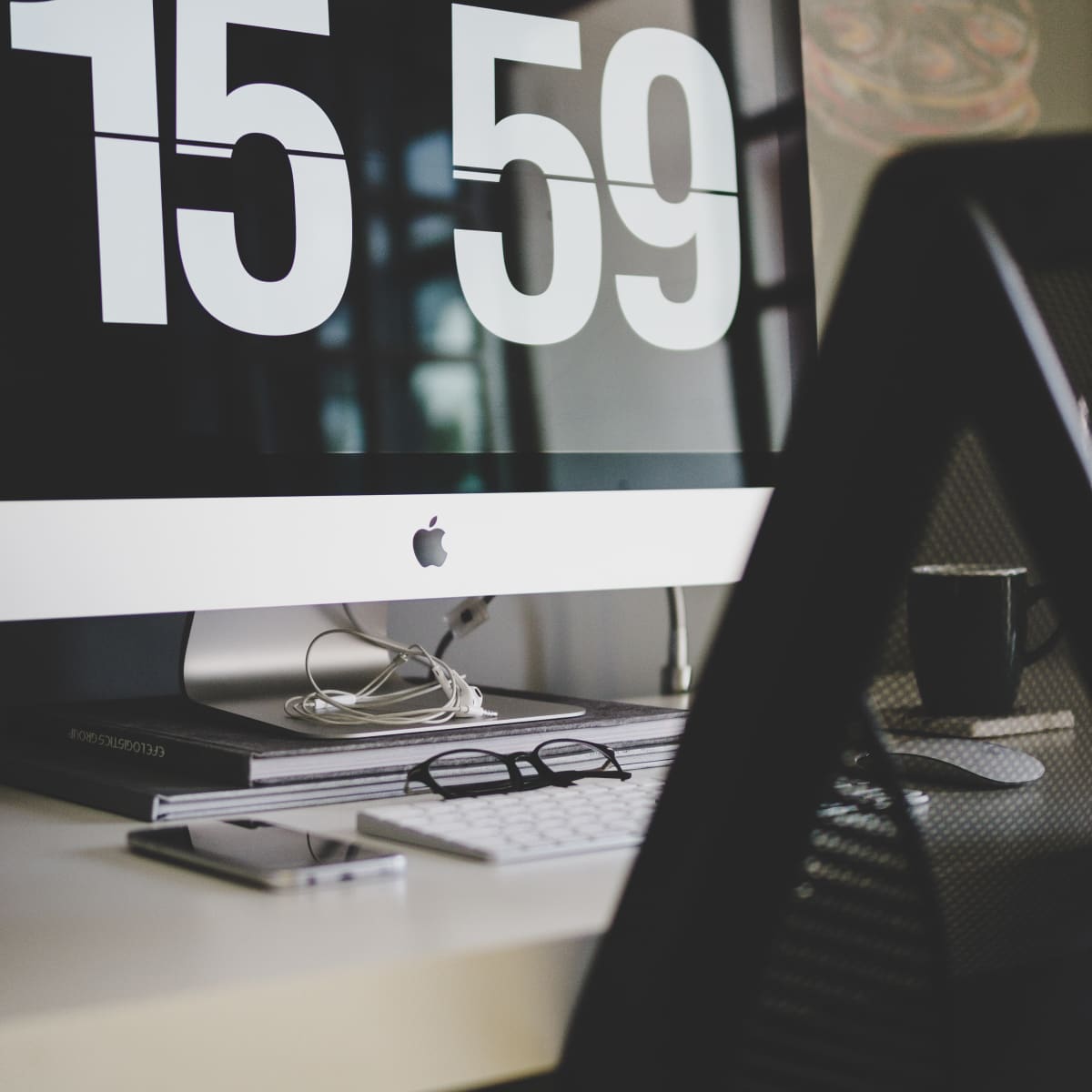The photograph depicts a meticulously organized workstation, characteristic of a clean, modern office environment. Dominating the scene is an Apple monitor with a sleek silver frame and a prominent black Apple logo. The monitor displays a minimalist screensaver featuring a black background and white numerals in the retro style of old alarm clocks, where the numbers flip over to change. 

The monitor rests on a stack of books atop an immaculate white desk. In front of the monitor, an Apple wireless keyboard is neatly positioned, accompanied by a pair of folded black-rimmed glasses. To the left of the keyboard lies an Apple iPhone, while to the right, a white mouse sits ready for use. A black coffee mug, placed on a white coaster, can also be seen on the right side of the desk. Beneath the monitor, a neatly arranged headphone cable adds to the orderly appearance.

The workspace also includes a standard office chair, featuring a mesh backrest with black rimmed support, which is pulled up tidily to the desk. The overall color scheme of the setup is predominantly black, white, and silver, contributing to the clean and efficient ambiance.